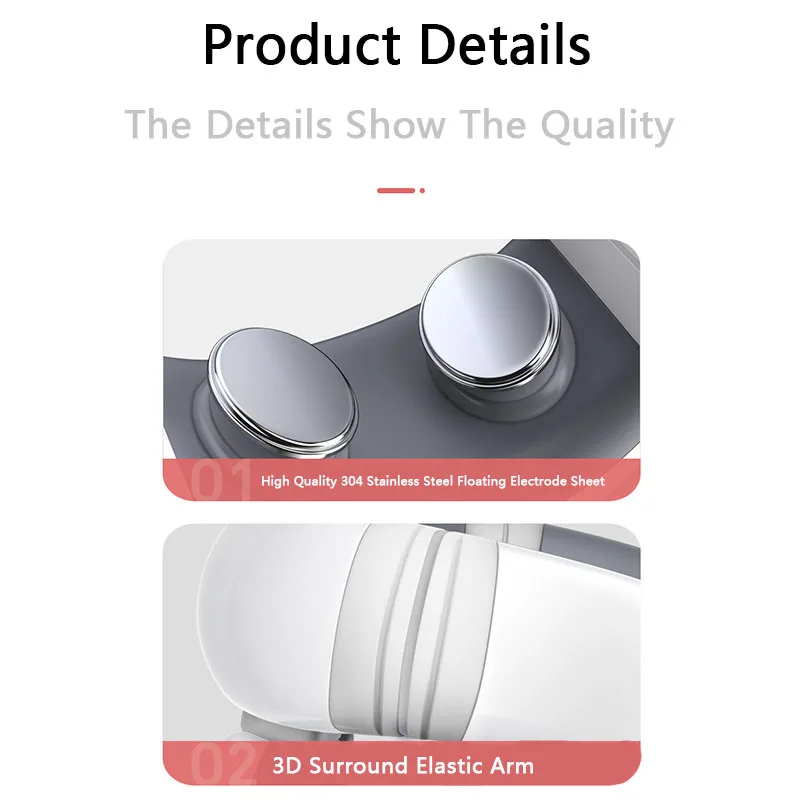"This is a screenshot of a minimalist website page focused on product details. At the top, the heading 'Product Details' is displayed in bold black lettering. Beneath it, in gray lettering, a subheading reads, 'The details show the quality.' A decorative horizontal line in peachy-red color with a dot at the end, resembling a horizontal exclamation point, separates the headings from the content below.

Following this, there are two images showcasing different components. The first image is a close-up view of two small, shiny, silver objects that resemble thumb sticks from game controllers attached to a curved material. It is labeled in the same peachy-red color as 'High quality 304 stainless steel floating electrode sheet.'

The second image provides a close-up of a plastic component, although the exact nature of the object remains unclear. This image is labeled as '3D surround elastic arm,' with matching peachy-red font.

The overall design of the website page maintains a simple and clean aesthetic, highlighting the detailed descriptions of the products."